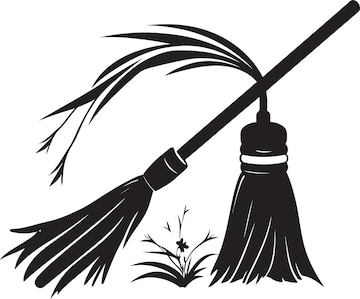The image is a black and white clip art illustration featuring two vintage broomsticks set against a plain white background. The broomstick on the left has a long wooden handle and is angled at about 45 degrees. The broomstick on the right, which is more full, sits on the ground and has a distinctive bundle of wheat instead of a traditional handle, with the wheat bending towards the left. Situated between the two broomsticks is a small, black flower growing out of the ground. The entire illustration has a slightly flowy and whimsical quality, with the black drawing accented by touches of white for detail.